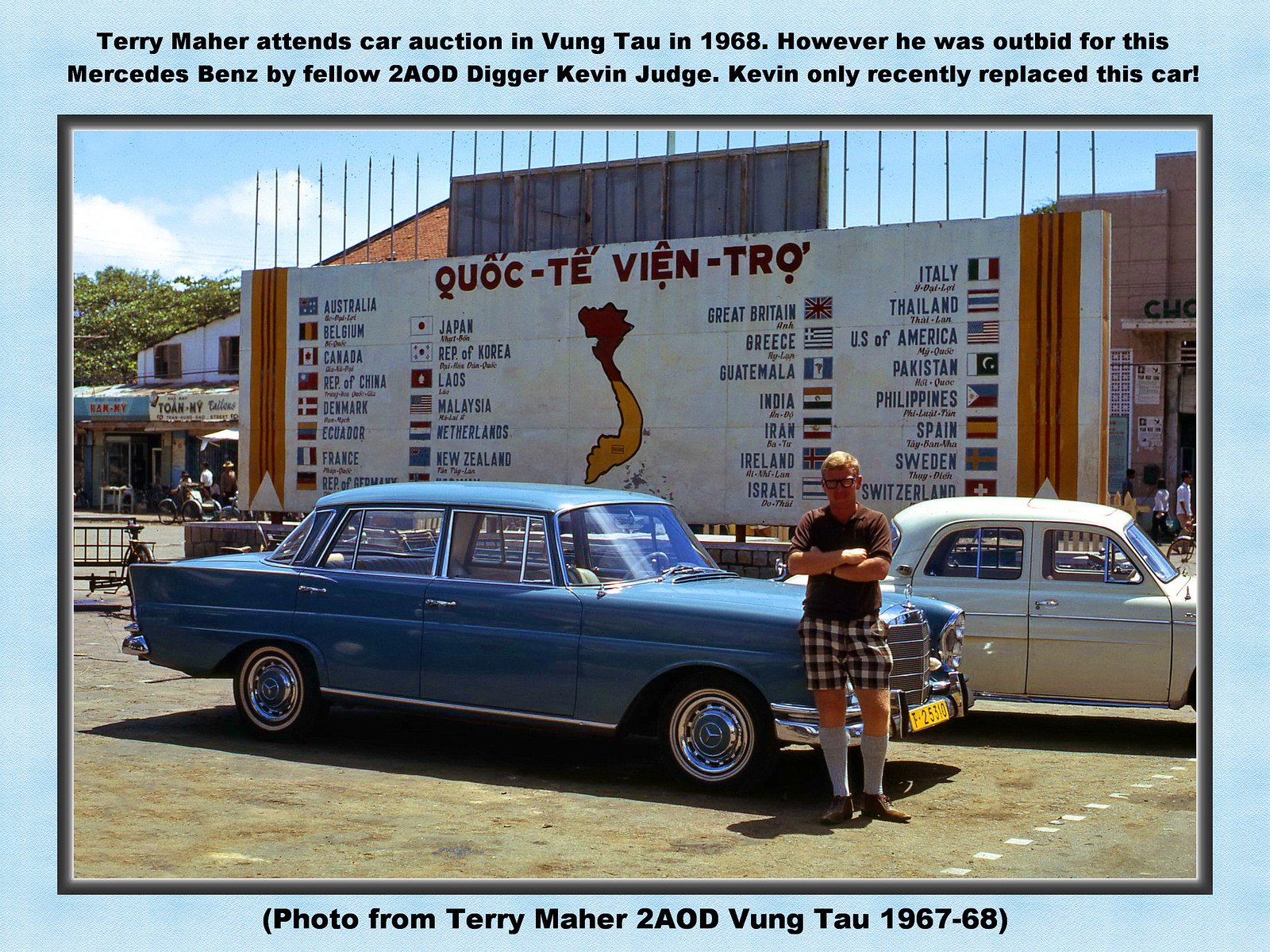Photograph taken in Vung Tau, 1967-68, featuring Terry Maher at a 1968 car auction. Despite his efforts, Maher was outbid for a beautiful, shiny medium blue, vintage Mercedes-Benz by fellow 2AOD digger, Kevin Judge, who recently replaced the car. Maher, standing tan and confidently posed with arms crossed, is dressed in a short-sleeved brown t-shirt, brown and white plaid shorts, gray high stockings, and brown shoes. The photograph is bordered with a light blue frame that encompasses a dark gray interior frame. Behind Maher and the Mercedes are another white car, a large map displaying numerous countries such as Australia, Belgium, and the United States, each with their respective flags, and a building in the distant background. This historical image is credited to Terry Maher from his time with 2AOD in Vung Tau during 1967-68.